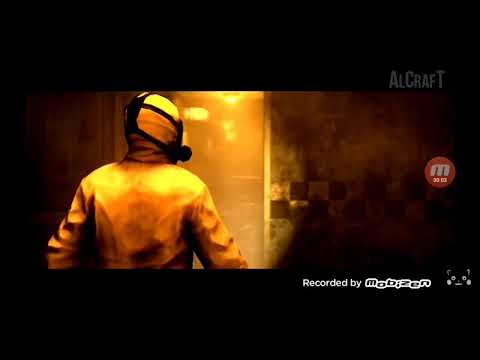The image portrays a person in a yellow hazmat suit turned away from the camera, their face obscured by a black hazmat mask. The setting appears to be indoors, possibly a bathroom, suggested by the white tiled walls with additional green or black tiling in the background. The image quality is somewhat blurry, contributing to an eerie and indistinct atmosphere. At the top of the image, the text "ALCRAFT" is displayed prominently in gray letters, with 'A,' 'C,' and 'T' standing out in uppercase while the other letters are smaller but still uppercase. The center features a red circular logo with the letter 'M' and some illegible numbers or marks below it. On the bottom left of the image, the text "recorded by Mobizen" is written alongside a small, stylized animal face with white eyes, ears, and mouth. The overall composition gives a sense of a possibly artistic or staged scene focusing on the mysterious figure and the associated cryptic elements.